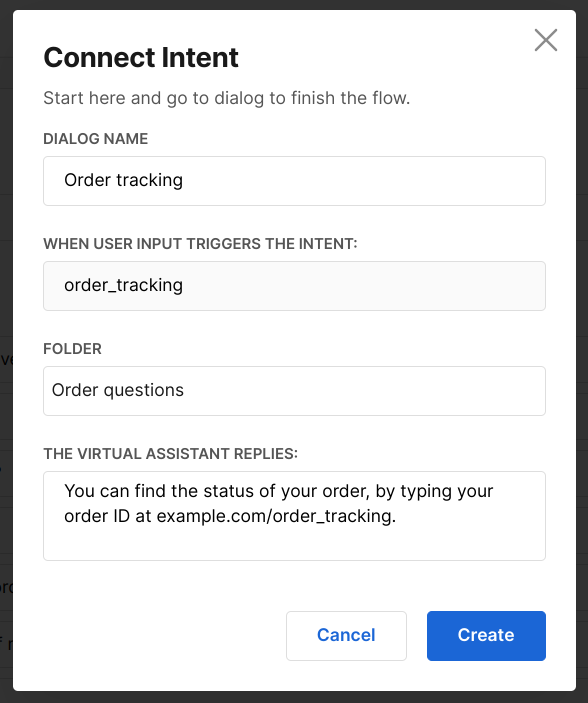The image displays a white pop-up window featuring various interactive fields and instructions for setting up a dialog flow. In the top right corner, there's a gray "X" button for closing the pop-up. The pop-up is titled "CONNECT INTENT" in bold black text on the left side, followed by instructions in gray text that read, "Start here and go to Dialogue to finish the flow."

Several input fields are present within the pop-up. The first field, labeled "DIALOGUE NAME" in all caps, contains the text "order tracking." The next section, titled "WHEN USER INPUT TRIGGERS THE INTENT," shows the input "order_tracking" in a lighter gray field, distinguishing it from the other fields.

Following this, there's a section labeled "FOLDER," with "Order Questions" entered in the corresponding field. Below it, under "THE VIRTUAL ASSISTANT REPLIES," the field contains the response text: "You can find the status of your order by typing your order ID at example.com/order_tracking."

At the bottom of the pop-up, two buttons are displayed. The left button is white with a blue outline and blue text that says "Cancel." The right button is blue with white text that says "Create."